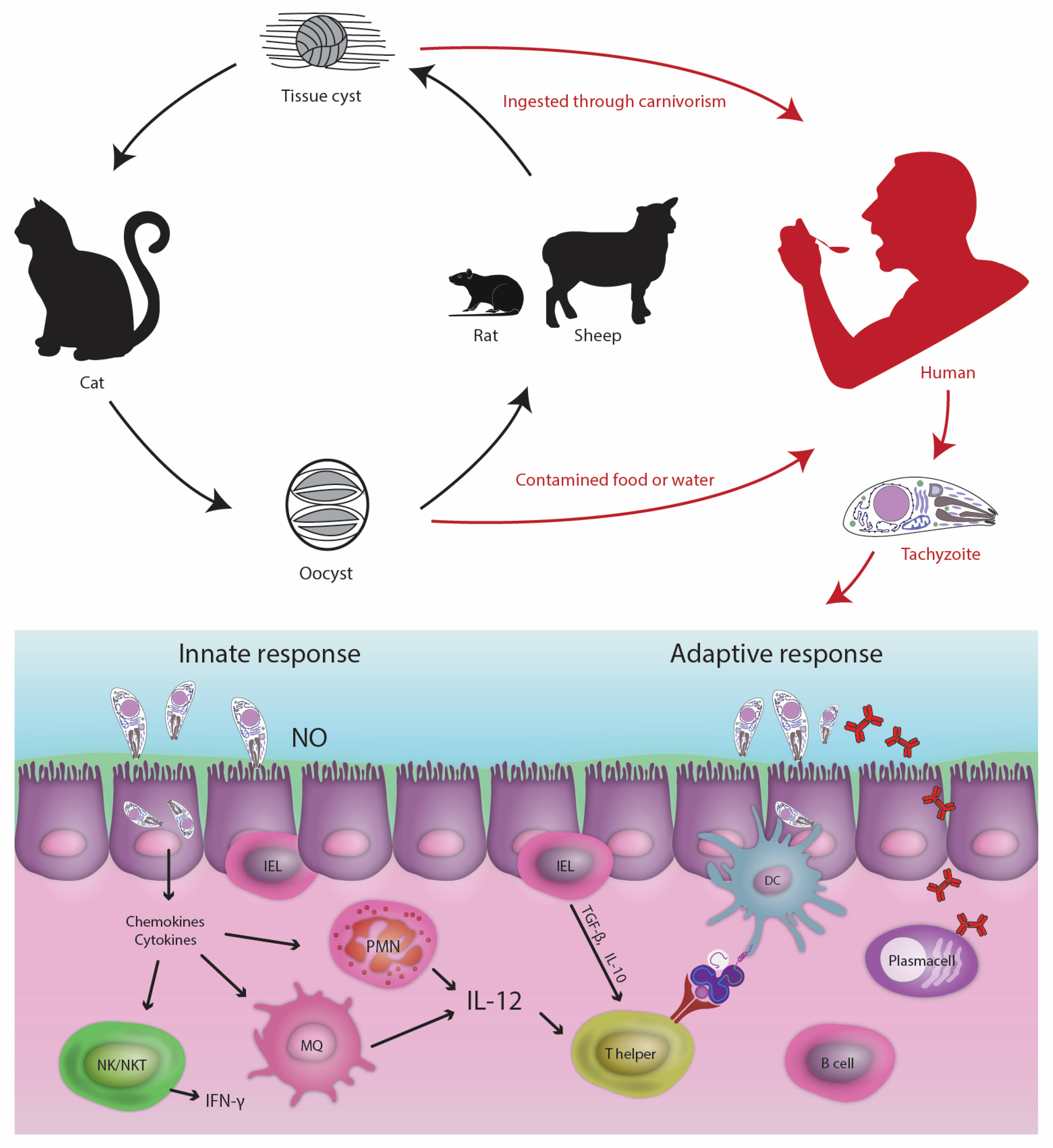This detailed illustration poster explains the transmission of disease from animals to humans, focusing on the food contamination process. The top half of the poster features a series of diagrams depicting a complex cycle, where contamination begins with animals such as rats, sheep, and cats. The arrows, varying in colors like purple, green, pink, and red, guide the viewer through the process. Black silhouettes of a rat and a sheep lead to an image labeled "tissue cyst," which is then connected to a cat, showing the progression of germs. From the cat, arrows point to "oocyst" and further to a human figure consuming food, illustrating how humans can get infected by either touching or ingesting contaminated food. 

At the bottom half, the poster transitions to a scientific depiction of how the disease affects human cells. It includes labels for "innate response" and "adaptive response" to show the immune system's reaction. The section is divided into a sky-blue top half and a pink bottom half, populated with various cellular illustrations. Purple, maroon, and other colored shapes represent different cell types and immune responses, including PMNs, MQs, and NKT cells, all identified with specific arrows and labels. The intricate visual design, with cartoon-like elements, uses floating objects, arrows, and detailed descriptions to convey the complex biological processes involved in the contamination and immune response.